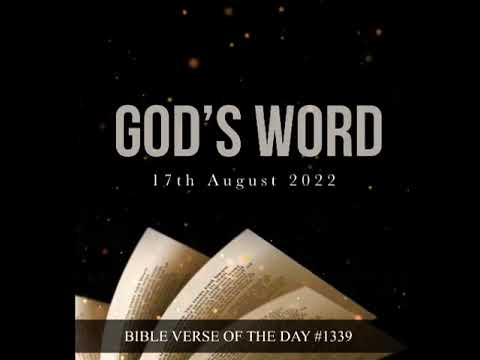The image appears to be a screen grab from a video, likely a podcast or a religious daily video feature. It has an almost entirely black background sprinkled with a few stars and planets, reminiscent of a night sky. In the foreground, there is white text that reads "God's Word" followed by "17th August 2022" in smaller text beneath it. Below this, the top of Bible pages are shown being flipped through, with visible black text on them. Overlaid on the flipping pages is a semi-transparent black bar with white text that reads "Bible verse of the day #1339."